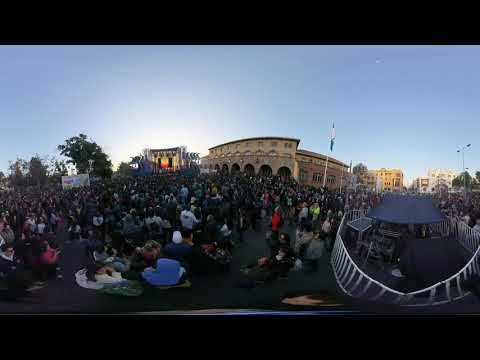The photograph captures a large crowd of likely thousands of people gathered outdoors in what appears to be a public square, around dusk. The scene features a warped, fisheye lens effect, that distorts the frame and creates a sense of enclosed chaos. Prominent in the background is a large building with multiple arches on its front facade, tinged with a dark gold hue from the setting sun, creating a light blue sky overhead. To the left, there's an elevated outdoor stage, complete with lights and large speakers, seemingly the focal point of the event. Trees also dot the left side of the scene, adding to the open-air atmosphere.

On the right side, there is a leaning white fence enclosure surrounding a small, navy blue tent or pavilion. The presence of a white and blue flagpole in front of a yellow and white building further to the right lends an official feel to the surroundings. The crowded foreground makes it hard to discern individual faces or clothing, adding to the sense of an immense, indistinct gathering. Overall, the image evokes the liveliness and somewhat chaotic ambiance of a large public event or festival.